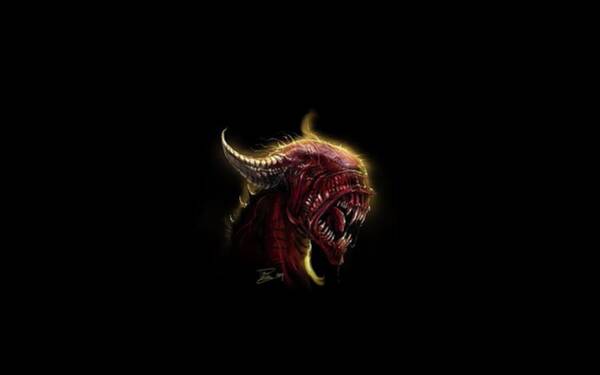The image showcases a detailed, computer-generated drawing of a monstrous creature's head prominently centered against a solid black background, creating stark visual contrast. The creature, depicted in a side view, emits a terrifying presence with its large, open mouth brimming with exceptionally sharp, long teeth and a prominent, big red tongue. Its skin, a shiny, leathery red, features intricate, strange patterning that adds to its unsettling appearance. The head, devoid of eyes and nose, is further accentuated by two horn-like protrusions that resemble long, pointy ears. A layer of flesh connects its massive mouth to the head, enhancing the creature's alien-like visage reminiscent of the monster from Ridley Scott's film. Surrounding the head is a golden glow that contrasts with the dark maroon, brown, yellow, and gold hues of the creature itself. Additionally, there appears to be a small, blurred white signature beneath the monster, further hinting at this being a piece of sci-fi digital artwork or a potential logo design. The extensive black void enveloping the scene emphasizes the intimidating central figure.